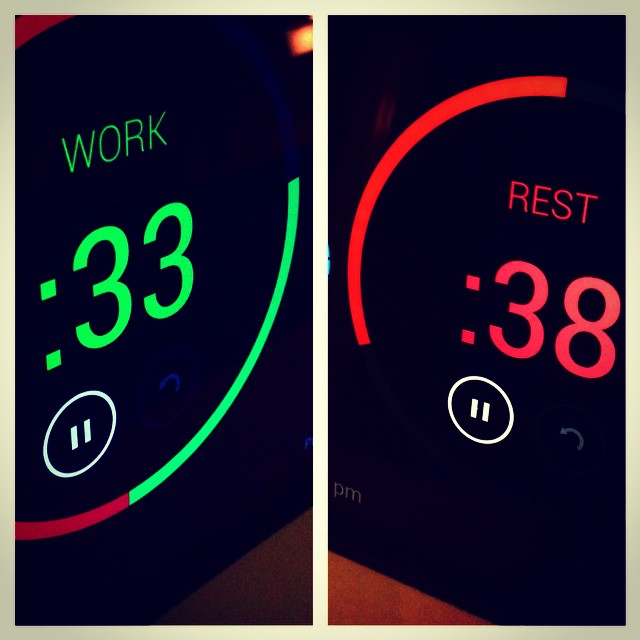This image depicts two digital stopwatches on a black device, illustrating different timing modes with vivid colors and clear screens. 

The device on the left displays a bright, neon green-colored "WORK" label in all capital letters. Below the label, the screen shows "33," likely indicating 33 seconds. The display is surrounded by decorative elements in blue, green, and red hues. Just underneath the 33-second display, there is a white pause button. Additionally, the left screen features a blue-lit arrow symbol, resembling a back or reset button.

On the right side, the same device showcases the label "REST" in bold red capital letters, against a backdrop of a red-lit circular frame. The screen prominently displays "38," which likely signifies 38 seconds of rest time. Similar to the left side, this display also includes a pause button below the seconds count, and features a white-lit arrow symbol.

Overall, the image captures a well-illuminated, multifunctional digital timer with distinct "WORK" and "REST" modes, distinguished by their respective green and red themes.